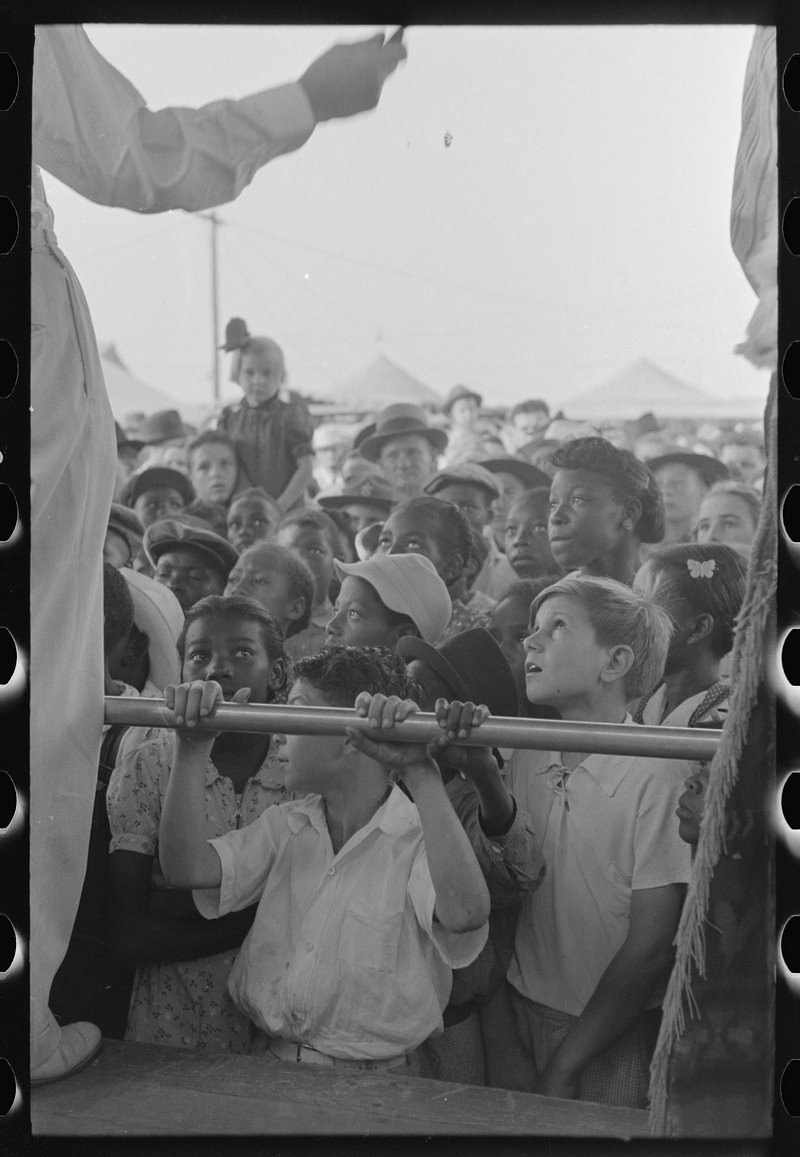In this vintage black-and-white photograph, a large gathering of children and a few adults, predominantly dressed in mid-20th century attire, are captured outdoors, all looking up attentively towards a man in an all-white suit standing on a platform. The man’s outstretched right arm directs their gaze towards the left side of the image, although more than half of his left side is cropped out. The children, a diverse group featuring numerous young boys and girls, are the primary focus, with one boy prominently holding onto a metal bar directly in front of the man on the stage. An adult wearing a bowler hat is visible among the children past the first few rows. The photograph exudes a sense of admiration and attention from the crowd, who are possibly responding to the man's speech. The backdrop includes a wide, faded white sky with cone-shaped white tents in the distance, further emphasizing the historic ambiance of the scene.